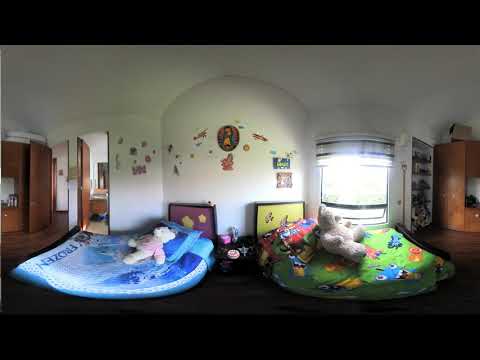The image is a panoramic photograph of a child's room that captures detailed and vibrant elements. The room features two small beds, each with distinct themes and decorations. On the right side, there is a bed with bright green sheets adorned with cars, a yellow headboard, and a large tan-colored teddy bear. This bed is placed next to a window set into a black frame with short black and white curtains, allowing sunlight to filter in and reveal hints of greenery outside. On the left side, there is a bed with a blue blanket branded with characters and colors from the Disney movie "Frozen," complete with the movie's title in blue text. This bed has a purple headboard and a white teddy bear with a red shirt resting on a blue pillow. Both beds are directly on the dark-colored floor and have various stickers and circle art adorning the white wall behind their headboards. The room further includes a brown door on the left and wooden shelving or bookcases on both sides.